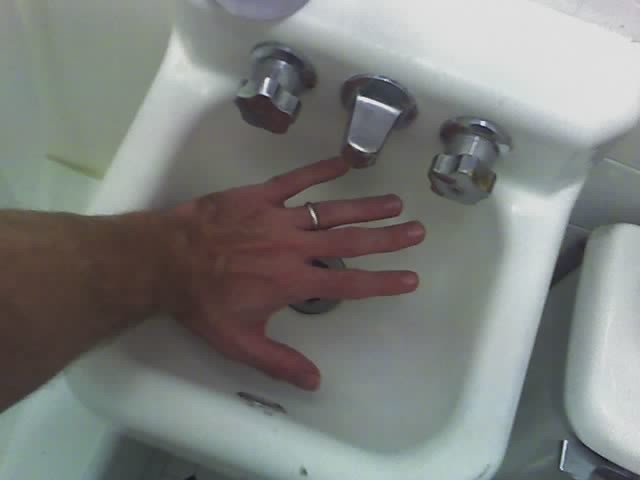This is a detailed, bird's-eye view photograph of a small, white porcelain sink with silver faucets and star-shaped knobs, characteristic of those found in public bathrooms. The image captures a left Caucasian hand, adorned with a silver wedding ring on the ring finger, spread out over the sink beneath the faucet. The hand's short, unpainted fingernails are visible, positioned centrally in the frame. To the right of the sink, part of a toilet tank and its handle are discernible. The faucet and its handles are short and stubby, contributing to the compact appearance of the sink. The photo, although slightly blurry, seems to be taken by the same person whose hand is in the image, giving a somewhat close-up and personal perspective. The hand is extended, emphasizing the sink's diminutive size, as the fingers nearly touch the sink's edges.